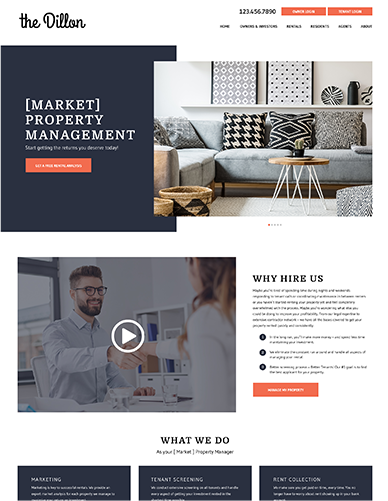The website for a company called "The Dylan" features a professional layout with a phone number displayed at the top, represented by placeholder text "1234567890." To the right, there are two prominent orange buttons, though their functions are unspecified. The main navigation menu includes categories like "Home," "Owners," and "Renters," suggesting the site is related to property rentals.

The focal point of the page is a beautifully styled living room with a pale blue couch adorned with graphic throw pillows. Above it, black-and-white framed artworks rest on a simple white shelf, complemented by a jug, pottery, and wicker items. The room features a white carpet, modern decor, and exudes a contemporary ambiance.

On the left side of the page, a slate-colored section reads "Market [Property Management]" with the subheading "Start getting the returns you deserve today." Below this, an orange button prompts users to "Get a Quote" or something similar.

Further down, there's a thumbnail depicting a man and a woman shaking hands, marked with a video play button. Adjacent to this is a section titled "Why Hire Us," followed by a descriptive paragraph and three numbered bullet points. Another call-to-action button appears beneath this segment.

Towards the bottom, there's a section labeled "What We Do" with three slate panels detailing services like marketing, tenant screening, and rent collection, accompanied by explanatory text.